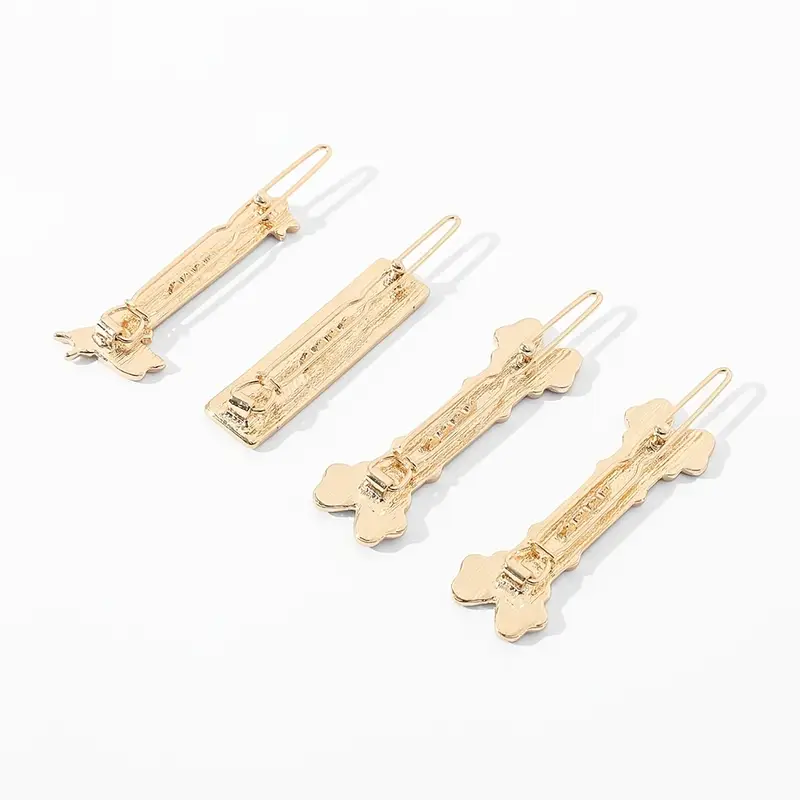The photograph showcases four gold hair barrettes, meticulously arranged diagonally on a pristine white background, with subtle shadows emphasizing their presence. Each barrette features a long clip that attaches to a small stud on one end and is fixed to a hinge on the opposite end. The design of the barrettes includes two with a distinct dog bone shape, a third that is a simple long rectangle, and a fourth, more elaborate piece that resembles a dog with a detailed head and a long body. Despite their artistic forms, all barrettes share a flat, metallic construction with prominent, elongated loops, giving them a polished yet puzzling appearance.